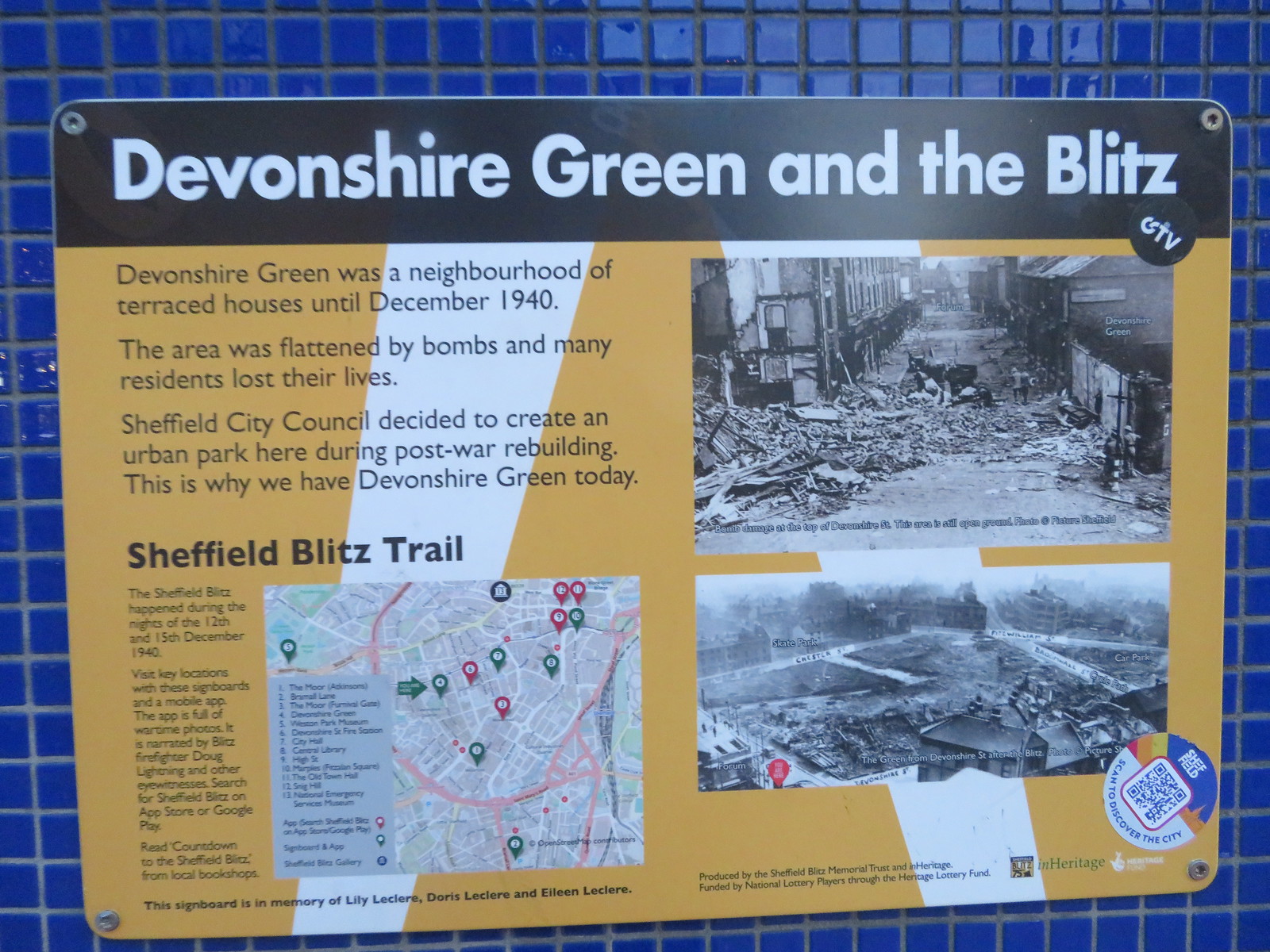The plaque mounted on a wall of blue tiles details the history of Devonshire Green and the Blitz. At the top, a black banner with white text reads "Devonshire Green and the Blitz." The upper left corner of the plaque narrates the tragic history: "Devonshire Green was a neighborhood of terraced houses until December 1940. The area was flattened by bombs, and many residents lost their lives. Sheffield City Council decided to create an urban park here during post-war rebuilding. That is why we have Devonshire Green today." Below this, in black letters, is the title "Sheffield Blitz Trail" followed by several paragraphs of additional context and an accompanying map with green and red markers. The right side of the plaque features two stacked black-and-white photographs depicting the devastation: one shows rubble and destruction, while the other captures a wider view of the cleared area after the bombing. A QR code is located at the bottom right of the plaque for more information. Circular stickers adorn the plaque, adding to the visual detail.